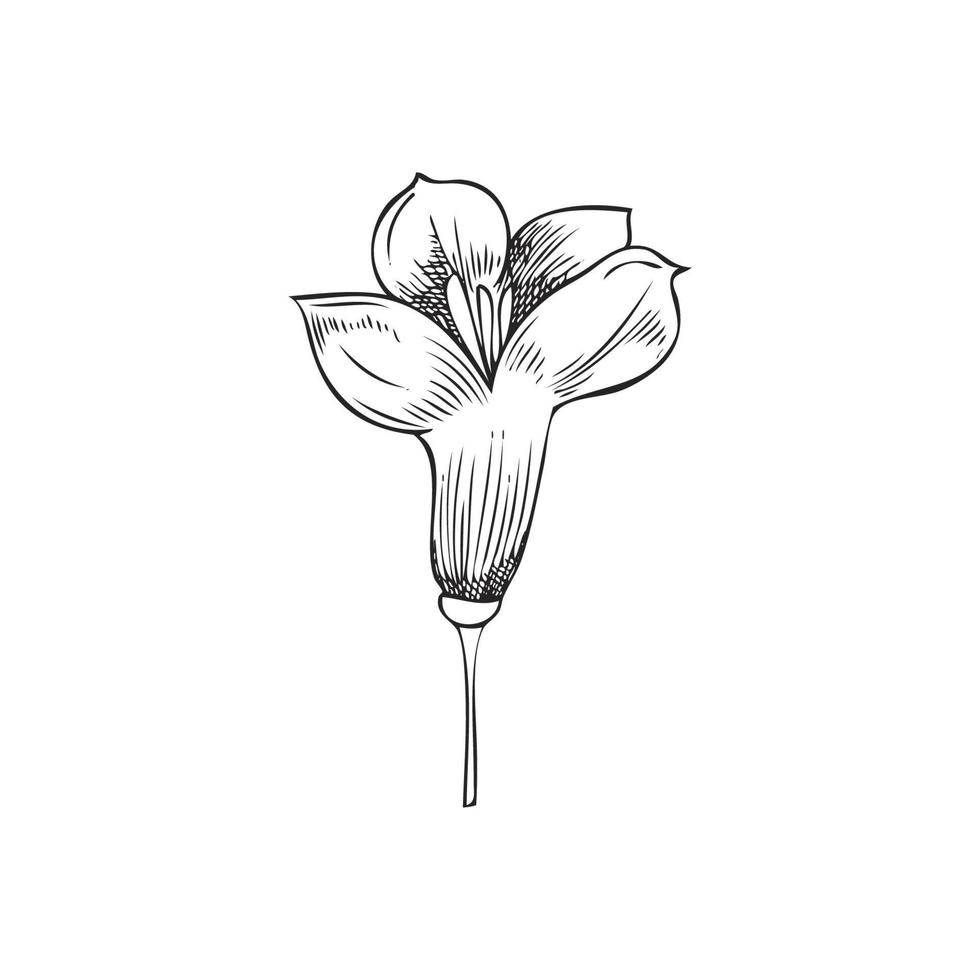This black-and-white drawing, possibly created with pen and ink, features a stylized yet unmistakably identifiable flower. Positioned against a completely white background, the flower's simplified design showcases a slender stem leading up to a cup-shaped or trumpet-like bloom. The flower consists of four petals, two of which are prominently in the foreground while two are visible at the back. A notable detail is that one of the petals on the right side intriguingly resembles the silhouette of a bird, complete with what appears to be a beak and eye. The center of the flower contains stamens extending outward, adding to its realistic detailing. To provide texture and dimension, crisscross hatching and vertical lines mimic shading throughout the petals, stem, and stamen. The overall effect is that of a refined doodle, displaying a balance between simplicity and thoughtful detail.